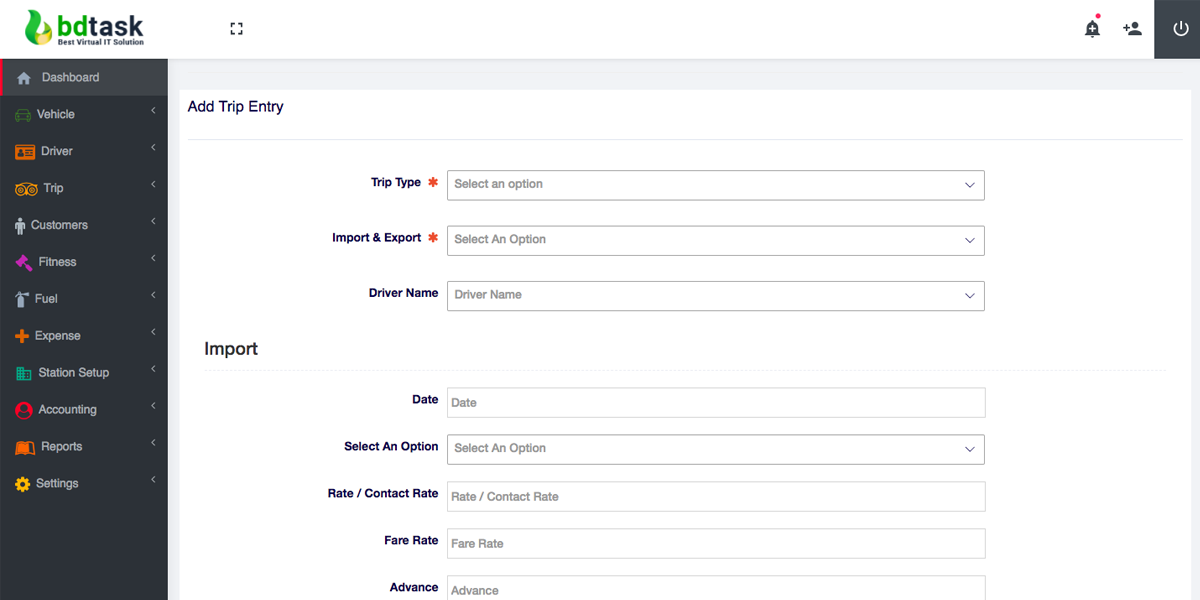The image depicts the front-end interface of an order management webpage named "BD Tasks - Best Virtual IT Solutions." The header of the webpage features a distinct white strip. On the left side of this strip is the text "BD Tasks" in green, followed by the slogan "Best Virtual IT Solutions" in black. Adjacent to the text is a small green flame icon with a yellow base.

Moving to the right side of the header, there are various icons: a bell with a plus sign and a small orange dot above it, a person icon, and what appears to be a power button symbolized by a circle with a strip on top.

Below the header, the majority of the screen is occupied by a white data entry box, which takes up about 80% of the interface. At the top of this box, there is a prompt in gray font that reads "Add Trip Entry." Further fields categorized as "Type Trip" with options "Import and Export," and "Driver Name" are available, each presented as a white drop-down box with gray text that says "Select an option."

Below the "Add Trip Entry" section is another rectangular section labeled "Import." This part includes several fields: date, select an object/option, rate, contract rate, fare rate, and advance, all of which are associated with white drop-down boxes.

To the left of the central data entry area is a black sidebar featuring various navigational icons with labels. The sections are listed as:

- **Dashboard:** Represented by a lighter black icon.
- **Vehicle:** No specific icon description provided.
- **Driver:** Icon resembling a driver's license.
- **Trip:** Icon resembling the owl symbol from TripAdvisor.
- **Customers:** Icon of a small person.
- **Fitness:** Icon resembling a judge’s gavel.
- **Fuel:** Icon resembling a tank.
- **Expense:** Icon with a plus sign.
- **Station Setup:** Icon depicting a building.
- **Accounting:** Icon with a person.
- **Reports:** Icon resembling an open book.
- **Settings:** Icon resembling a flower in a circle.

These sections, presented in various colors like orange, gray, purple, and pink, facilitate user navigation and data entry within the website, helping users manage trip and import-related information seamlessly.